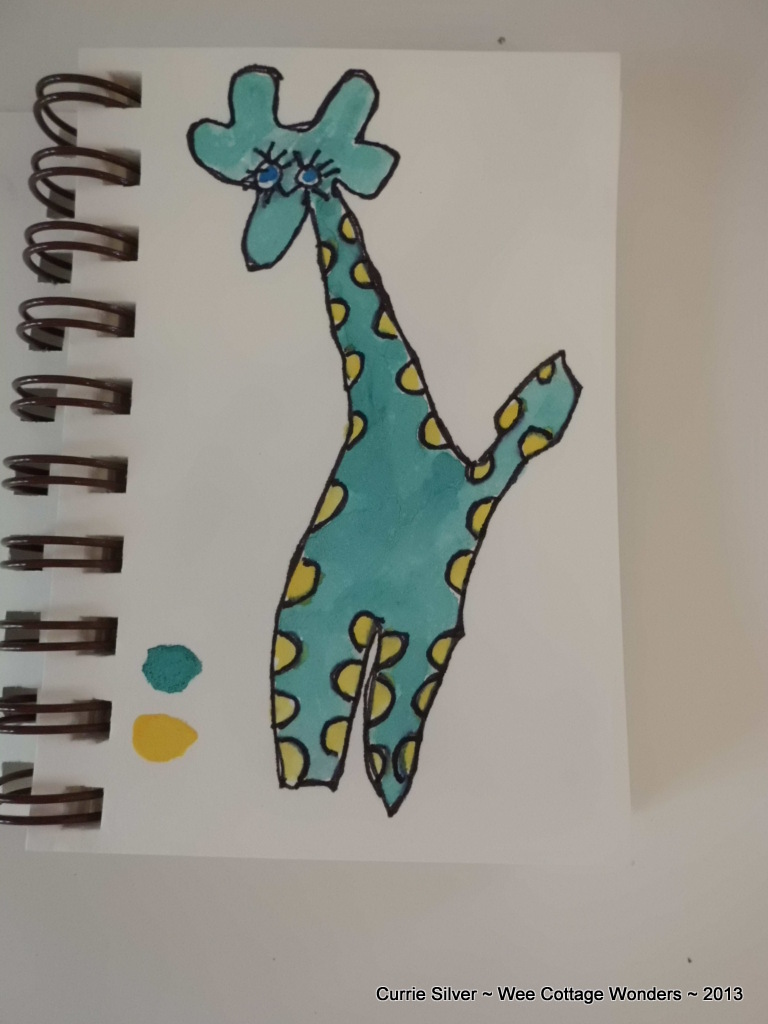The image shows a detailed, cartoonish sketch of a giraffe on a white piece of paper, which is part of a pocket-sized, ring-bound notebook. The sketch features a blue or light blue giraffe with big blue eyes and prominent eyelashes. The giraffe's head is angled up and to the left, sporting two small bumps on top and ears that point outward. Its neck is long, and the body is decorated with light orange, almost yellow, spots primarily along the periphery, including the neck and both inner and outer legs. The giraffe's tail, short and pointed up to the right, adds to the whimsical nature of the drawing. The drawing is executed in watercolor, with possible outlines in black ink or crayon. At the bottom left corner of the page, below the giraffe, are small circles colored in yellow and green, and to the far bottom left, adjacent to the giraffe, are blue and light orange paint marks. The notebook's black spiral binding is visible on the left side of the paper.